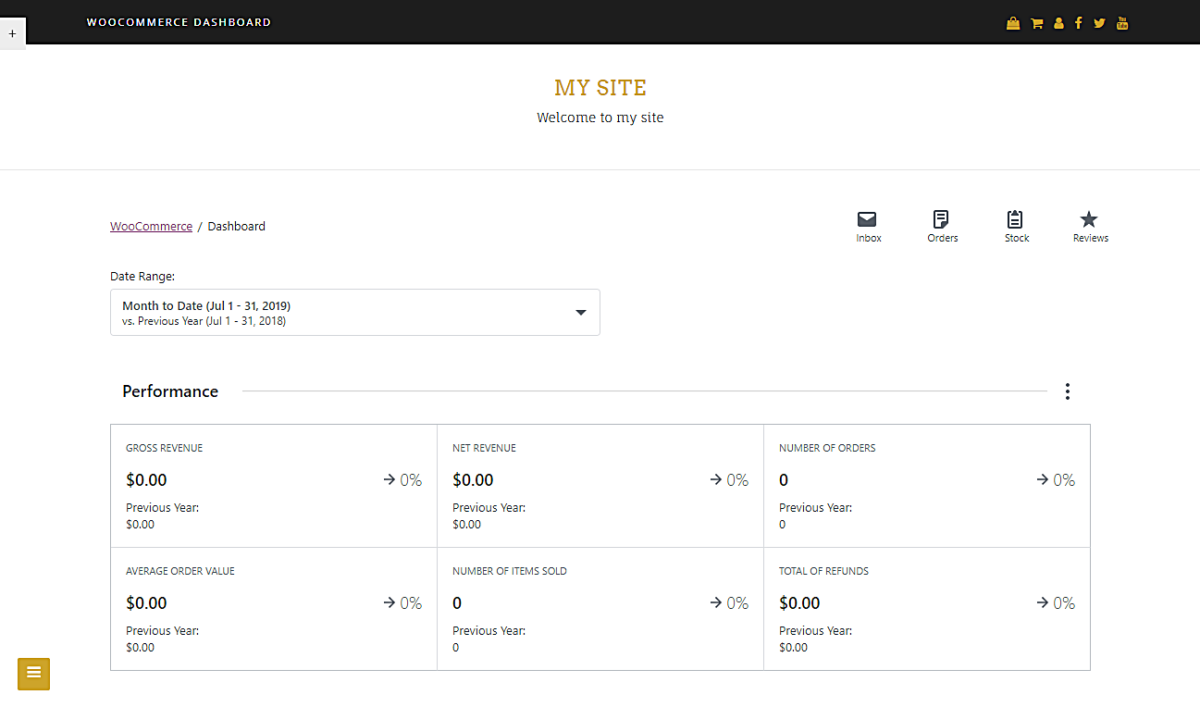Screenshot Description of a WooCommerce Dashboard Website:

The image is a screenshot of a WooCommerce Dashboard web page, featuring a predominantly white background with black text. At the top of the screenshot, there is a black menu bar with white text that reads, "WooCommerce Dashboard." On the far left of the menu bar, a gray square with a plus sign button is visible. On the right side of this menu bar, there are several gold-colored icons including a briefcase, a shopping cart, a user logo, as well as icons representing Facebook, Twitter, and YouTube.

Beneath the menu bar, the white background continues and displays the text "MY SITE" in capital letters and gold font centrally. Directly underneath that, in black text, it reads "Welcome to My Site." To the right-hand side of the webpage, there are four icons representing an inbox, orders, stock, and reviews, each for easy access to those sections.

The main content area of the dashboard showcases a date range drop-down menu, which currently has the range from July 1st to July 31st, 2019 selected. The dashboard provides detailed performance measures divided into six categories: Gross Revenue, Net Revenue, Number of Orders, Average Order Value, Number of Items Sold, and Total Refunds. Each category presents specific metrics to give a comprehensive overview of the site's sales performance for the selected date range.